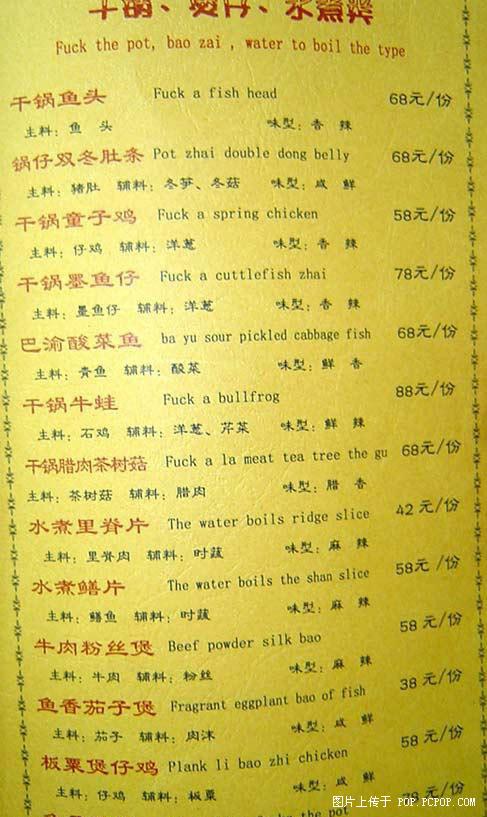The image depicts a vertically-oriented rectangular menu, featuring a textured yellow background. The texture is evident with visible lines, wrinkles, and scratches, creating a nuanced surface that reflects light in varying degrees, giving the appearance of depth and dimension. The menu appears to be from a foreign country, evidenced by the presence of numerous symbols resembling Chinese characters framing its border. The border design includes a repetitive floral pattern.

At the top section of the menu, there are red symbols written in a foreign language, followed by an unconventional English text that reads, "F the pot, bao zai, water to boil the type." Continuing downward, the menu alternates between red and black symbols, interspersed with English translations. Phrases such as "F a fish hand" appear repeatedly amidst these symbols. Additionally, the menu lists numbers like "68" beside the symbols, suggesting item numbers or prices.

In the bottom right corner of the menu, a set of white symbols are present, alongside a website address, providing further information or online access to the menu's offerings.